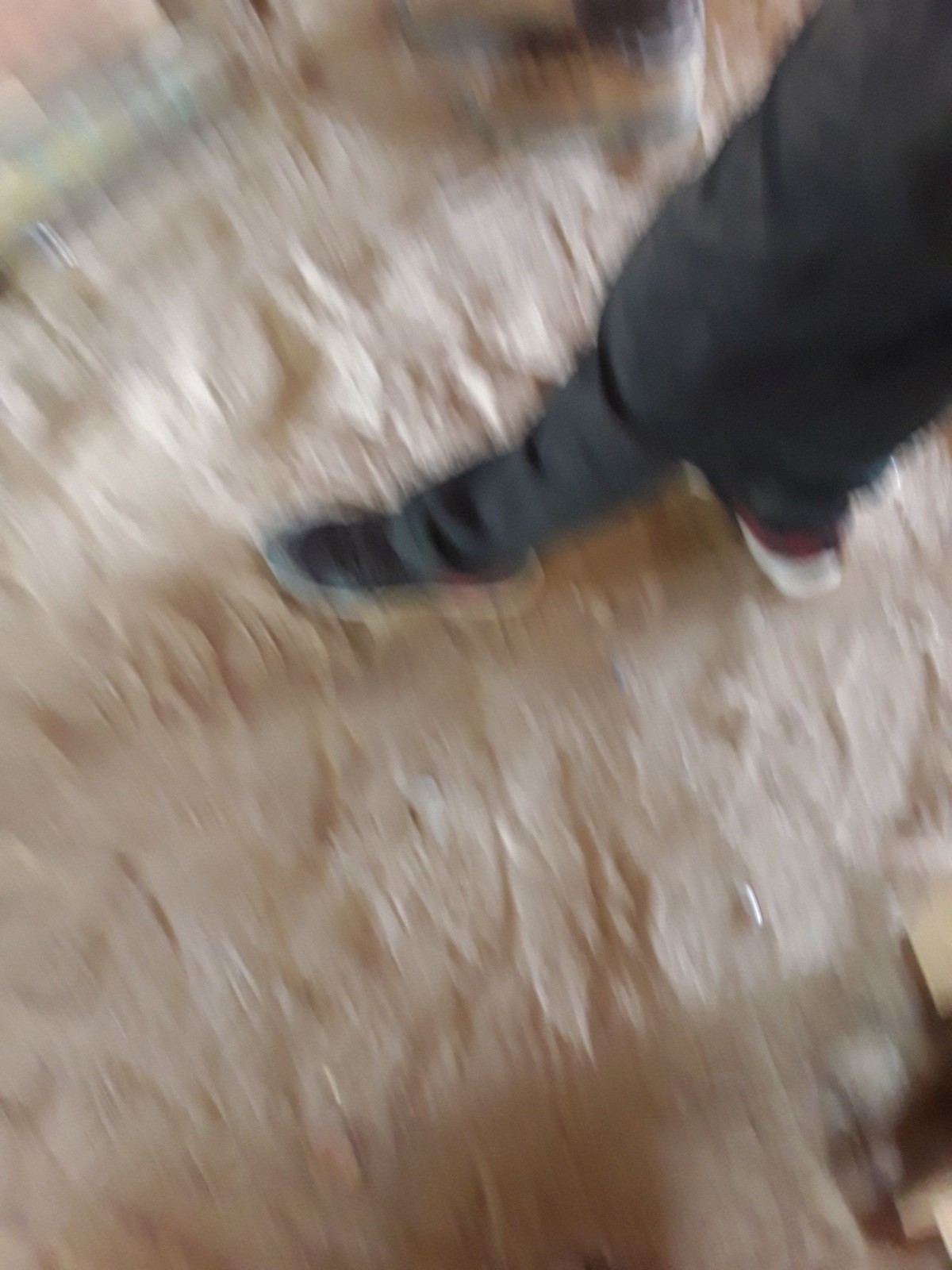This image features a blurred and out-of-focus scene with an uneven white floor that appears textured and inconsistent. Starting from the top right corner, a figure can be discerned standing and extending downward toward the left corner. The individual is dressed in a long black t-shirt, black pants, and black shoes accented with red details and white soles. One of his feet is pointed upward while the other is directed to the left. His arms, clad in a striped long sleeve, partially hang down from the top.